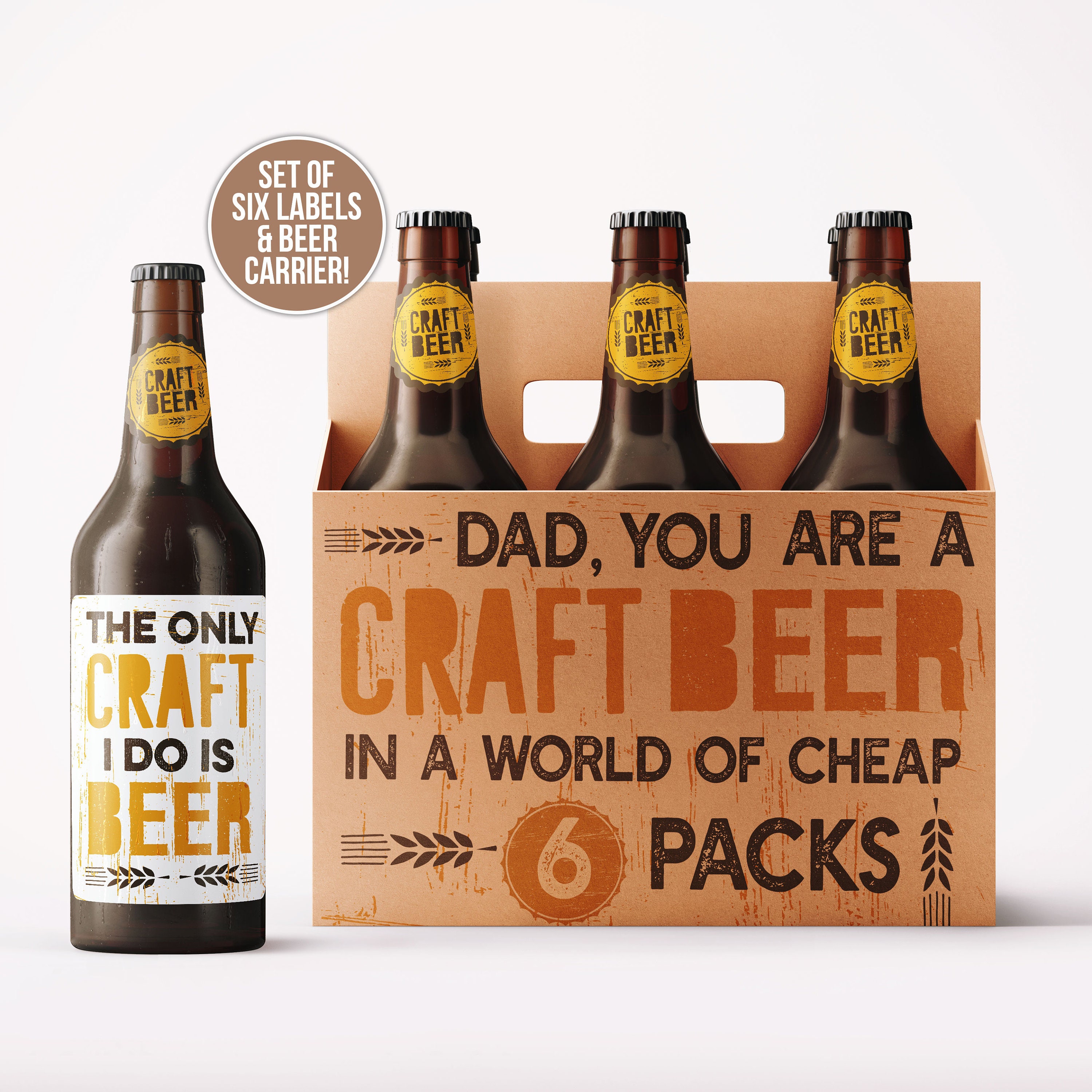A mock-up of a craft beer features a prominent display of a single beer bottle and a pack of six bottles. The solitary bottle, with a distinctive yellow sticker at the top reading "Craft Beer," is positioned beside the six-pack. The bottle's label clearly states, "The only craft I do is beer" against a white background. The six-pack, made from a light orangish-brown material, has black and orange text that reads: "Dad, you are a craft beer in a world of cheap six-packs." Each of the dark brown bottles within the pack has a matching yellow sticker at the top. Between the single bottle and the six-pack is a decal detailing that the set includes six labels and a beer carrier. The design also incorporates drawings of barley, adding a traditional brewing element to the packaging.